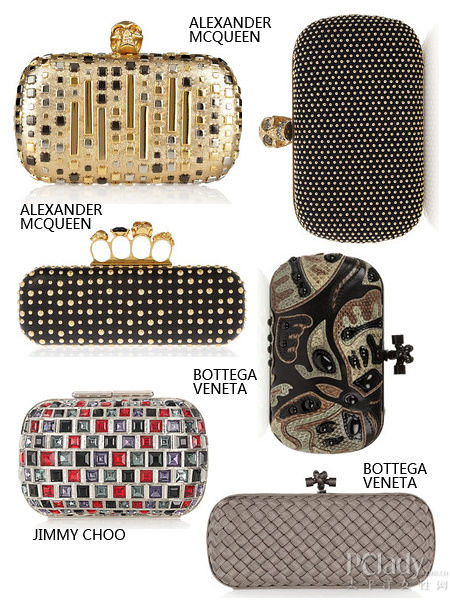This image displays a selection of six high-end designer clutches against a clean, white background, which gives it a pristine, art-studio feel. Starting from the top left, the first clutch is a luxurious gold piece by Alexander McQueen, adorned with square studs and a unique face resembling a skull with monkey-like features. To its right is another Alexander McQueen clutch, this one black, embellished with small gold studs in a polka dot pattern and featuring a bedazzled version of the same distinctive face. Below the first gold clutch is another black Alexander McQueen piece, this time with larger and smaller gold studs, and designed with four rings meant for fingers, resembling brass knuckles.

On the top right is a stylish Bottega Veneta clutch with a sleek black exterior dotted with white embellishments. Below it is another Bottega Veneta creation, showcasing a sophisticated black design with gray and brown swirling patterns made to mimic a woven texture. Finally, the bottom right features a beautiful Bottega Veneta clutch with a gray crisscross pattern that almost looks woven.

The bottom left side flaunts a vibrant Jimmy Choo clutch bejeweled with purple, black, and gray square studs. Each piece is not only a testament to the impeccable design and craftsmanship of these luxury brands but also a striking demonstration of both elegance and artistry in miniature handbags.